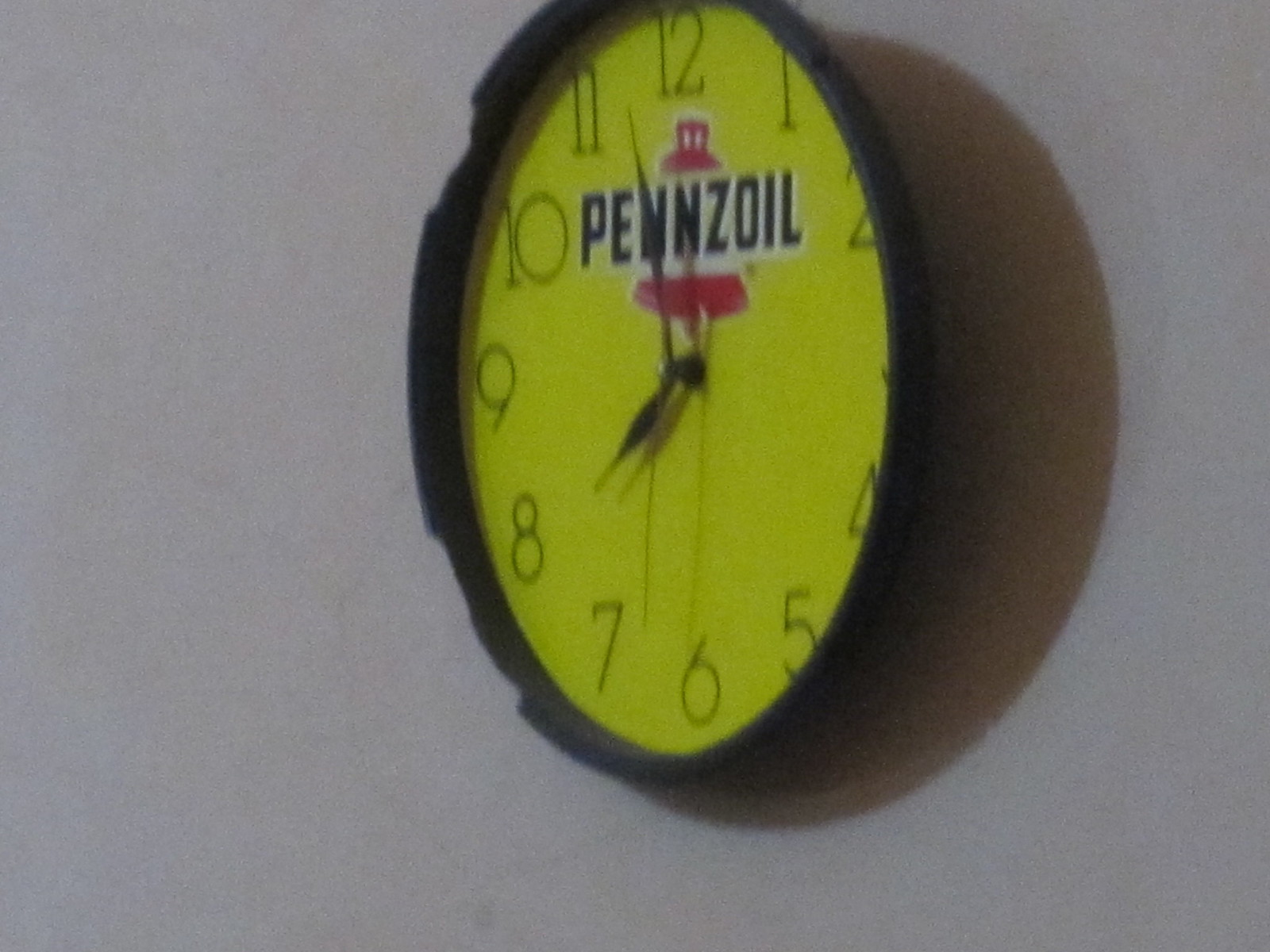In this photograph, a circular analog wall clock with a black frame is prominently featured against a white wall. The clock's face is yellow, encircled by a somewhat chipped black rim. The numbers on the clock are black and arranged in the usual 1-12 sequence for analog clocks. At the top under the number 12, there is a logo with the word "Pennzoil" in black letters, outlined in white, set against a red bell-shaped icon. The clock has simple black hands for hours and minutes, along with a thin, black seconds hand, showing the time to be around 7:57. A shadow, resembling a crescent moon, is cast on the wall behind the clock, adding to the image's depth. This clock, likely made of cheap plastic, seems suited for a mechanic's office, reinforcing its branding as an oil-sponsored item.